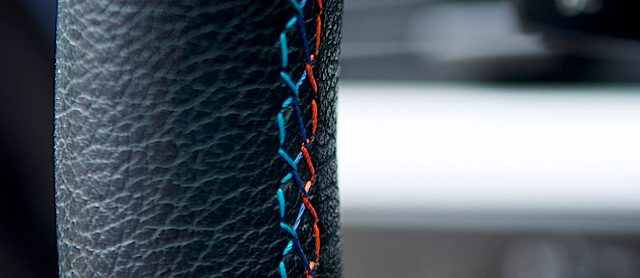This is a highly detailed close-up photograph of a textured black pleather surface, possibly a steering wheel cover, showcasing its leathery grain and intricate stitching. The focused area to the left reveals vertical, slightly irregular stitching in reddish-orange, dark blue, and light blue threads, forming a semi-zigzag pattern. This stitching appears to secure the cover, hinting that it may be reinforcing the pleather. To the right of the image, the background is blurred, with a horizontal white streak that could be interpreted as a vehicle's windshield, surrounded by darker elements in shades of black and gray. The combination of the sharp, textured pleather with the vibrant, crisscrossing threads against a blurred backdrop creates a visually striking composition.